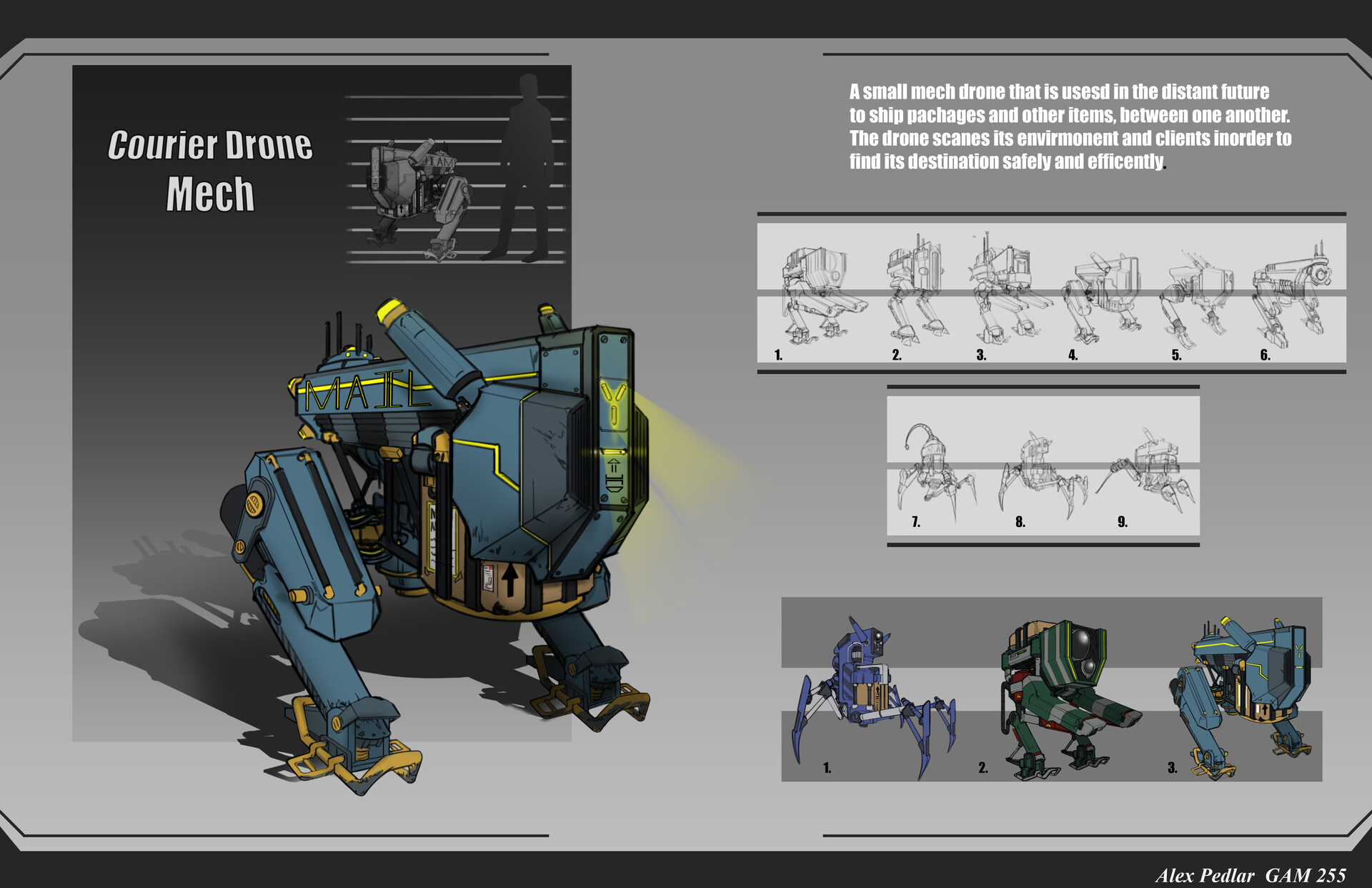The image is a detailed diagram of a futuristic mechanical drone titled "Courier Drone Mech" in the upper left corner. It features a dark blue tank-like machine with legs, labeled "male" on its side. Above this tank, there's a grayscale depiction of a smaller tank beside a silhouette of a person. The background of the image is gray, bordered by black. In the top right corner, a description reads, "A small mech drone that is used in the distant future to ship packages and other items. The drone scans its environment and clients in order to find its destination safely and efficiently."

Furthermore, the image includes a series of numbered sketches arranged in two rows, with steps numbered 1 through 6 demonstrating the development and operational sequence of the drone. Below these rows, there are three additional sketches numbered 1, 2, and 3, showing the refined stages of the drone's design. In the bottom right corner, there are three colored illustrations of different drone models: a purple spider-like machine, a blockier gray and green machine, and another resembling the initial blue tank labeled "male." Lastly, the bottom right corner bears the text "Alex Peddler GAM255."